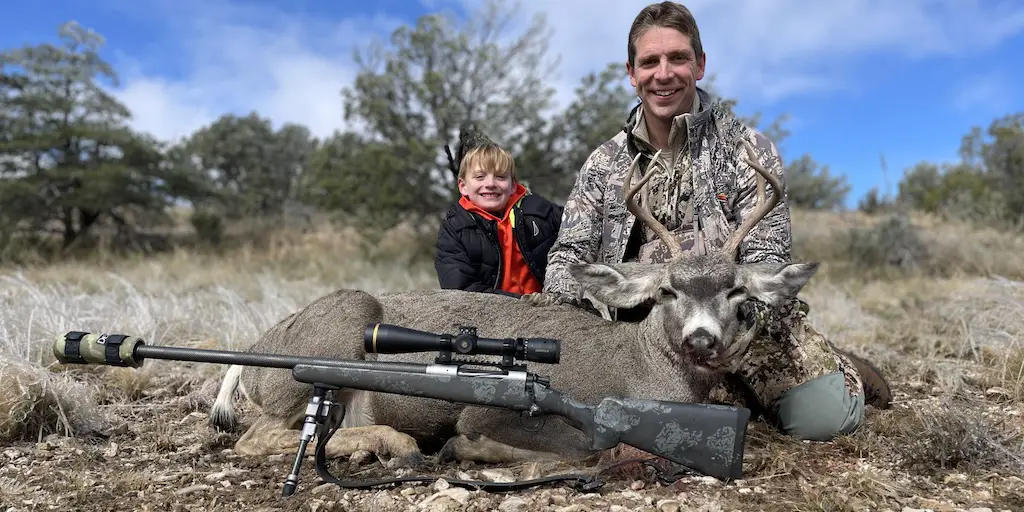This outdoor photograph depicts a man and a small child posed behind a recently shot deer, set against a backdrop of blue sky and white clouds with distant trees along the horizon. The terrain is a dry grassland with stringy grey-brown grass and scattered sagebrush. The man, dressed in a camouflage jacket, blue jeans, and brown boots, is holding up the deer's head, which features light gray antlers. The deer, lying on its side, shows gray fur with white markings around its ears and above its nose. At the man's left is a smiling child with blonde hair, wearing a black jacket over a red shirt, visible only from the waist up. In front of the deer, a rifle is positioned with its butt under the deer's head and a black scope and cylindrical piece at the barrel's end. The ground beneath them is dotted with dirt and rocks. Both individuals appear pleased with their hunting success, adding a mix of pride and somberness to the scene.